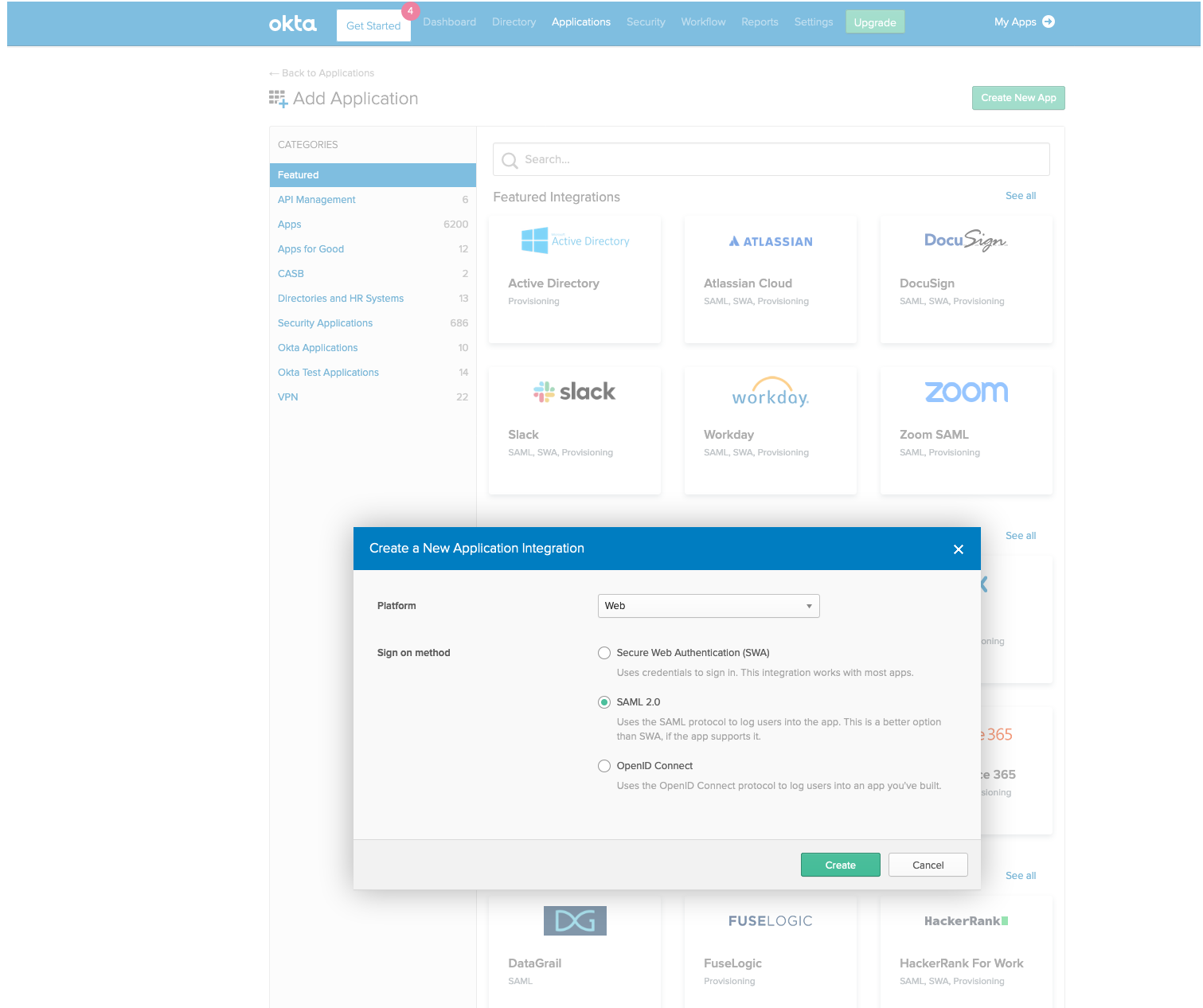The image displays a desktop screenshot of a web-based application or software tool named "Okta." The interface features a menu bar across the top, with the "Get Started" option highlighted in white and blue text. There are four notifications indicated by a notification symbol next to "Get Started." 

The top menu includes options such as Dashboard, Directory, Applications (which appears to be highlighted), Security, Workflow, Reports, Settings, and Upgrade. To the right, there is a link for "My Apps" with an accompanying right-facing arrow. 

Below this main menu, there are actionable buttons labeled "Back to Applications," "Add Application," and "Create New App." The system offers a range of options for application types, including:
- API Management (5 options)
- Apps (6,200 options)
- Apps for Good (12 options)
- CASB (2 options)
- Directories and HR Systems (13 options)
- Security Applications (686 options)
- Okta Applications (10 options)
- Okta Test Applications (14 options)
- VPN (22 options)

A search bar allows the user to find "featured applications" such as Active Directory Provisioning, Atlassian Cloud, DocuSign, Slack, Workday, and Zoom, each with descriptions of their functionalities or use cases.

A pop-up window titled "Create a New Application Integration" includes a prominent blue button for creating a new app integration. The pop-up can be closed by clicking a white 'X' in the corner. The "Platform" option is set to "Web" through a drop-down menu. Under the "Sign-on method" section, three options are listed:
- Secure Web Authentication (SWA): Uses credentials to sign in, suitable for most apps.
- SAML 2.0: Uses the SAML protocol for login, recommended if the app supports it (this option is currently toggled on).
- OpenID Connect: Utilizes the OpenID Connect protocol for logging users into custom-built apps.

At the bottom of the pop-up, there are two buttons for confirming or canceling the action, labeled "Create" and "Cancel," respectively.

The overall interface suggests that this tool is designed for managing various applications and integrations, likely used for business or work-related purposes.